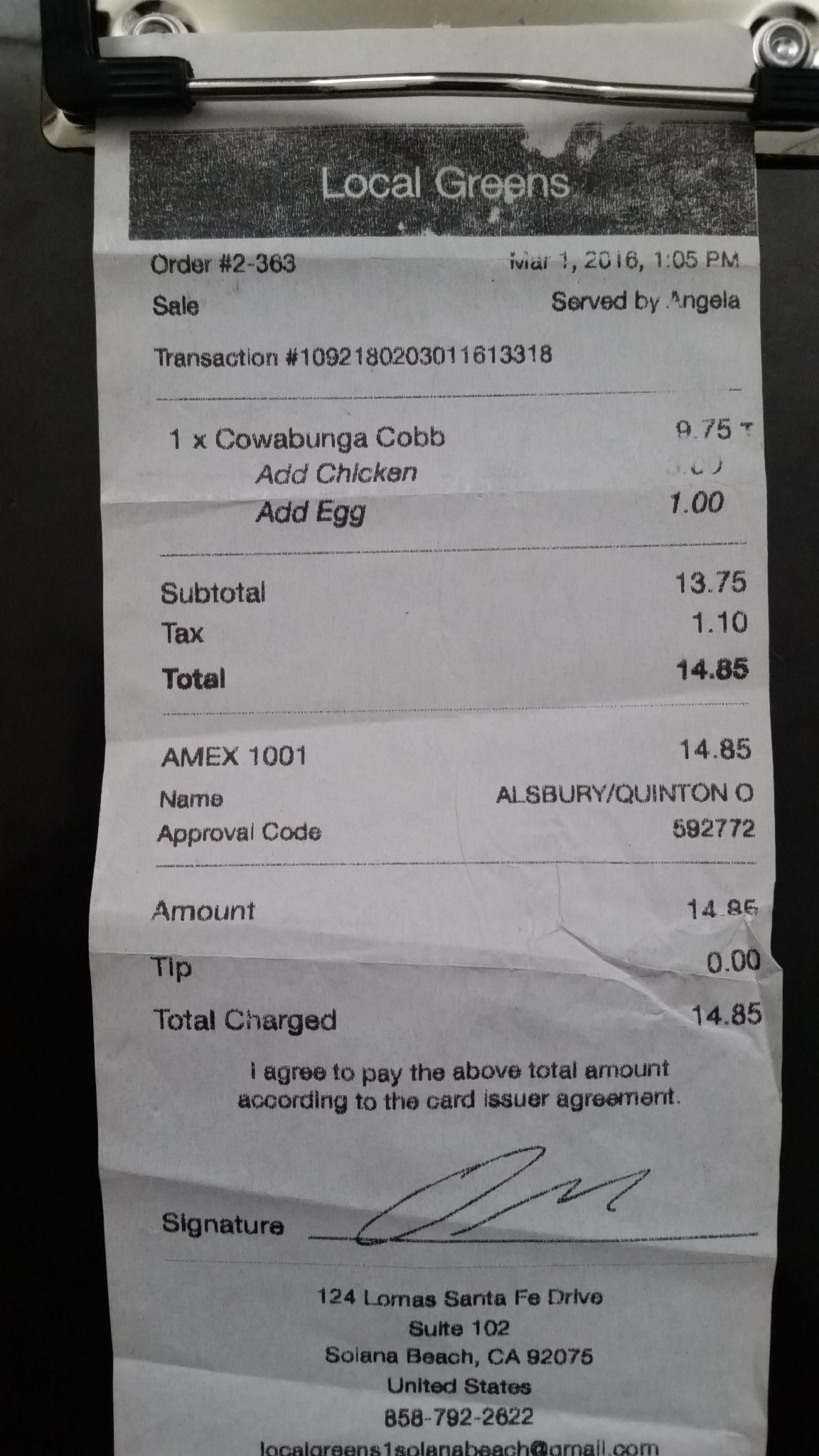A close-up image features a dark, solid black background that contrasts with a metallic object prominently placed in the center. The focal point includes a black rectangular label adorned with crisp white text. The label reads "Order Number: 2-363" in bold, clear font. Below, additional details in a similar white text indicate the sale transaction specifics: "Served by: Angela" and "Transaction Number: 10921803." The image effectively highlights the essential information related to the order and transaction, rendered against the stark backdrop for emphasis.